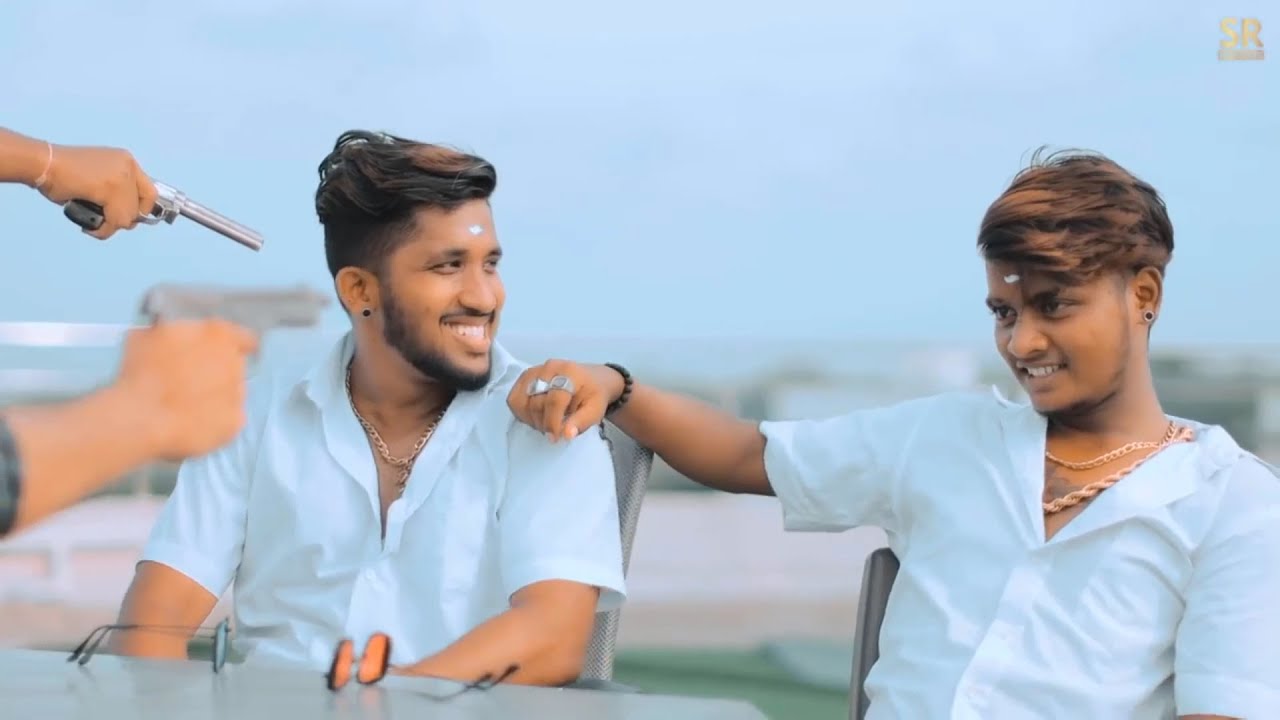In this playful and staged outdoor scene, two men are seated in chairs facing the camera against a blurred backdrop of a grey-blue sky. Both men are dressed similarly in light blue button-down short-sleeved shirts and gold chains around their necks. The man on the left sports dark, brownish hair, shaved sides, a mustache, and a beard. He also wears a black earring and has grey dots in the middle of his forehead. This man is turning towards the man on his right, who has black hair with hints of brown or red, wears an earring, a bracelet on his right hand, and two rings on his first and middle fingers. His hand rests on the shoulder of the man on the left. In front of them is a table with two pairs of sunglasses, one reflecting orange and the other blue. To the left of the scene, two outstretched arms hold guns pointed at the seated men, adding to the whimsical, prop-like nature of the photograph. Both men are smiling and laughing, contributing to the light-hearted atmosphere of the image.